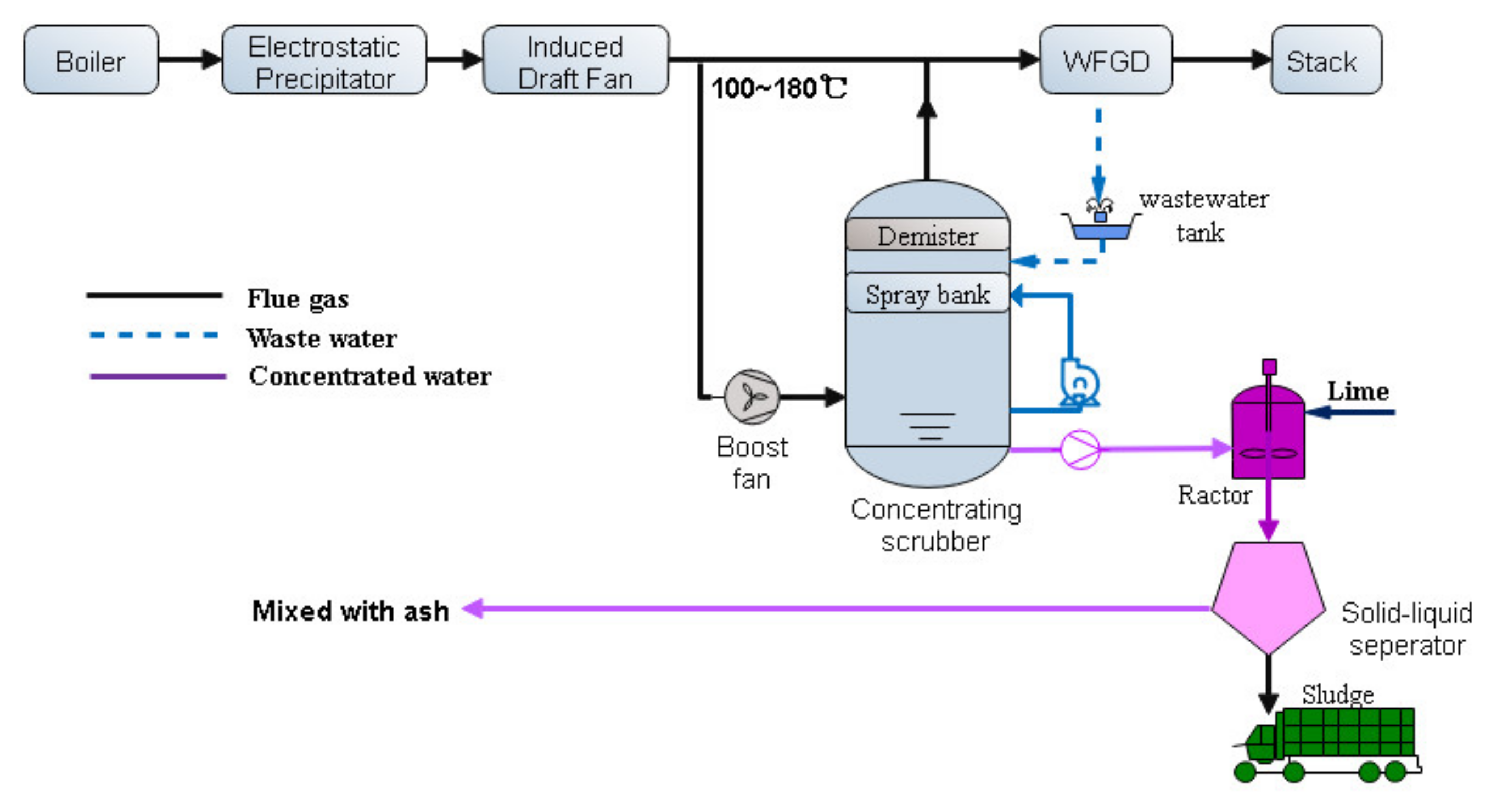The diagram illustrates a detailed flowchart of an industrial process, beginning at the boiler located in the upper left corner. The process sequence is indicated by various arrows: starting with a black arrow for the flue gas that moves to the electrostatic precipitator, followed by the induced draft fan, and leading horizontally to the WFGD (Wet Flue Gas Desulfurization) unit. The flow continues to the stack where the gases are released. Additionally, the diagram features a demister and spray bank as part of the intermediate steps, enhancing the scrubbing efficiency. Below this, the system incorporates a boost fan and a wastewater tank.

A color-coded legend on the far left explains that the black solid line represents the flue gas flow, the blue dotted line indicates wastewater, and the purple line denotes concentrated water flow. The wastewater treatment process is detailed further by the inclusion of shapes and symbols for the concentrating scrubber, lime reactor, and the solid-liquid separation unit, which ultimately converges into the sludge that mixes with ash. This sludge is represented as going into a green dump truck at the end of the process. The diagram also incorporates light blue panels labeling key components such as the boiler, electrostatic precipitator, induced draft fan, WFGD unit, and wastewater tank, providing a clear and comprehensive view of the interconnected stages.